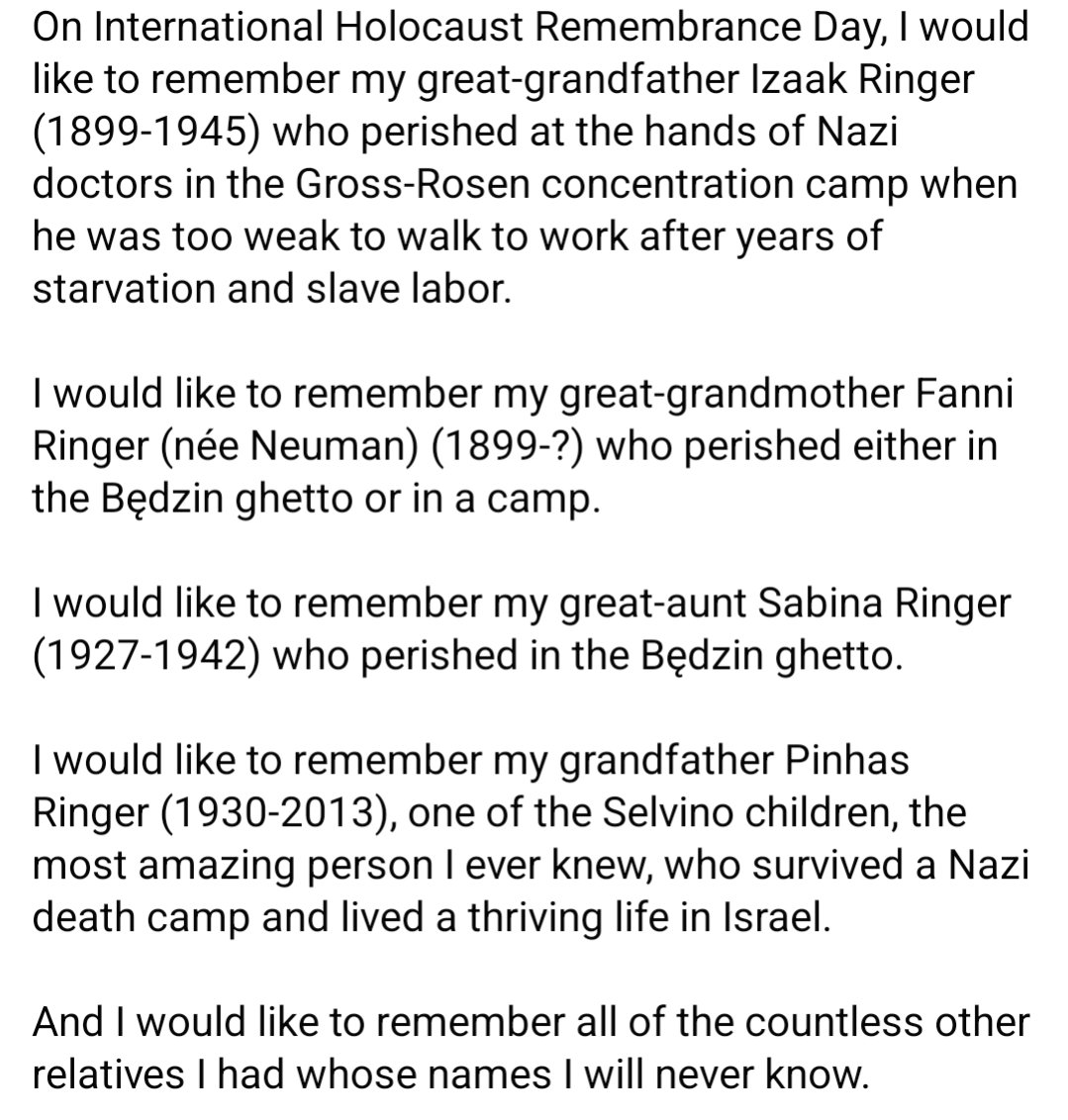On International Holocaust Remembrance Day, I would like to remember my great-grandfather, Isaac Ringer (1899-1945), who perished at the hands of Nazi doctors in the Gross Rosen Concentration Camp when he was too weak to walk to work after years of starvation and slave labor. I also honor my great-grandmother, Fanny Ringer (née Newman, 1899-unknown), who perished either in the Bedzin Ghetto or a camp. I would like to remember my great-aunt, Sabina Ringer (1927-1942), who perished in the Bedzin Ghetto. My grandfather, Pinhas Ringer (1930-2013), one of the Selvino children and the most amazing person I ever knew, survived a Nazi death camp and lived a thriving life in Israel. Finally, I would like to remember all of the countless other relatives I had whose names I will never know.